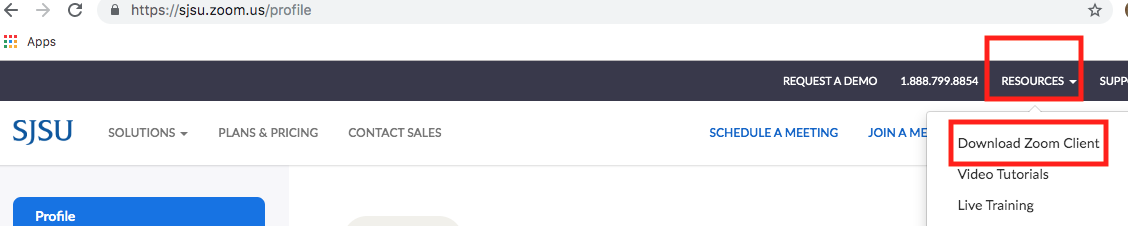The screenshot showcases a website interface with various navigation and informational elements. 

At the very top of the image, a web browser's navigation bar features the conventional back arrow, forward arrow, and refresh icon, all shaded in gray. The address bar displays the website's URL and includes a grayed-out star icon on the right, typically used for bookmarking.

Below the address bar, a gray navigation bar spans the width of the page, adorned with white text. This bar highlights options like "Request a Demo," a contact phone number, and the word "Resources," which is encased in a red rectangle. Further below, three more options are listed in gray text: "Download Zoom Client," "Video Tutorials," and "Live Training," with "Download Zoom Client" also highlighted by a red rectangle.

On the left side of this gray navigation bar, in bold blue uppercase letters, is "SJSU." Next to it, gray text lists additional navigation items: "Solutions," "Plans and Pricing," and "Contact Sales." To the right of these options, blue links read "Schedule a Meeting" and "Join a Meeting."

Further down, a blue bar features the word "Profile" in white text. The image appears to be cropped at this point, as a horizontal line indicates a cutoff, with the space below rendered entirely in white. 

The overall composition of the screenshot provides a clear glimpse of the website's navigational structure and user interface elements.